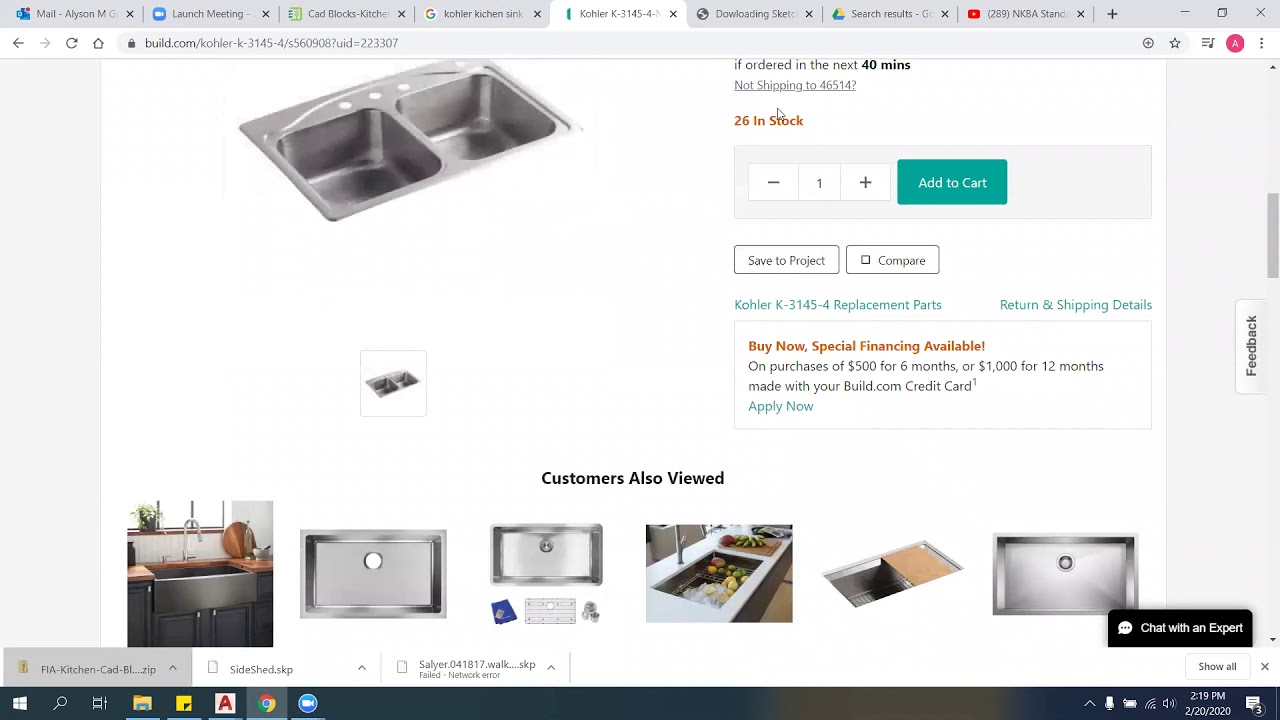Screenshot of a product listing on a website showcasing a double stainless steel kitchen sink. The product name is partially obscured, but the listing highlights urgent ordering with a note saying "Order in the next 40 minutes." The shipping information indicates it is not available for the ZIP code 46514. The listing shows 26 units in stock and includes options to increase or decrease the quantity, add the item to your cart, compare it with other products, or proceed directly to purchase. There is also a promotion for special financing available: for purchases over $500, 6-month financing is offered, and for purchases exceeding $1,000, 12-month financing is available, contingent upon using a bill.com credit card.